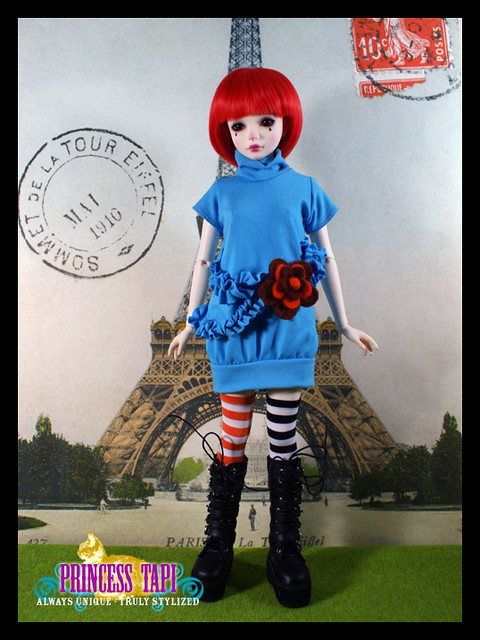In the foreground of the image stands an intricately styled doll with short, vibrant red hair and long bangs obscuring part of her dark eyes. The doll's face is adorned with striking makeup, including very little red lips and what appears to be dark tears streaming from her eyes, evoking a melancholic expression. She is dressed in a knee-length, short-sleeved blue sweater with a cowl neck, cinched at the waist by a blue sash embellished with a prominent red flower. Her legs are clad in contrasting tights—red and white stripes on the left leg and black and white stripes on the right leg—complementing her tall, intricately laced black boots that rise to just below her knee. In the background, a postcard-like image of the Eiffel Tower is set against a grassy field, bordered in black. The top right corner of the image features a red stamp with a black emblem, while the left side displays a thin black seal inscribed with "Somet de la Tour Eiffel, March 1910." The bottom left corner of the image bears the text, "Princess Tappy, Always Unique, Truly Stylized."